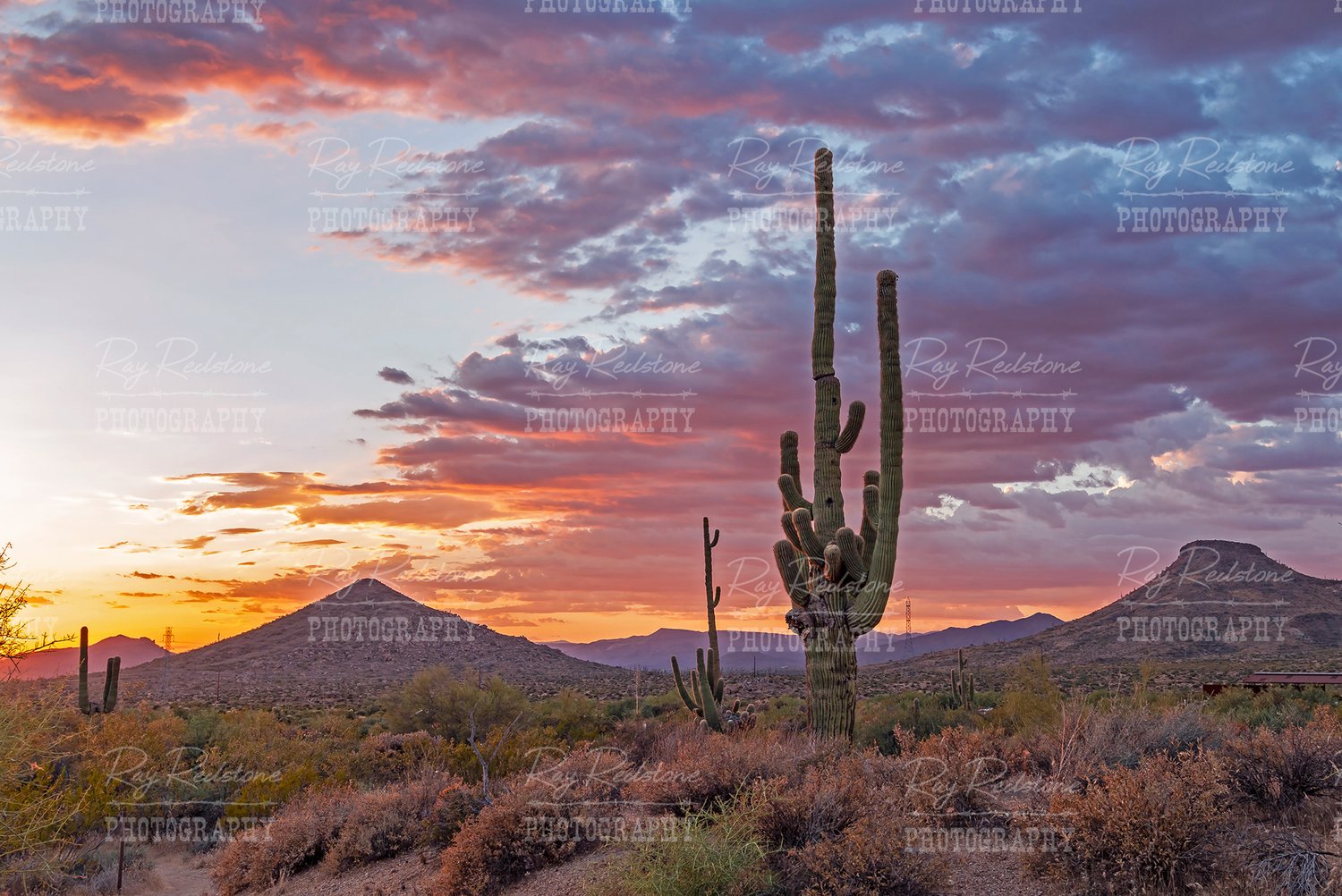A horizontal color photograph titled "Desert Serenity," captured by Ray Real Stone Photography. The watermark, styled in vintage typography, subtly traverses the image, adding a touch of authenticity. This professional photograph showcases a breathtaking desert landscape adorned with towering saguaro cacti dispersed across the sandy terrain. At the base, a mixture of brown, brushy vegetation and light green plants add depth and contrast. In the distance, textured mountain ranges rise against the horizon, adding a rugged backdrop. The sky, painted with the vibrant hues of sunset, features a striking orange strip near the horizon, seamlessly blending into an array of pink, yellow, blue, and purple clouds that stretch horizontally across the scene. The cacti stand out vividly in shades of green and dark green, harmonizing with the serene palette of the desert evening.